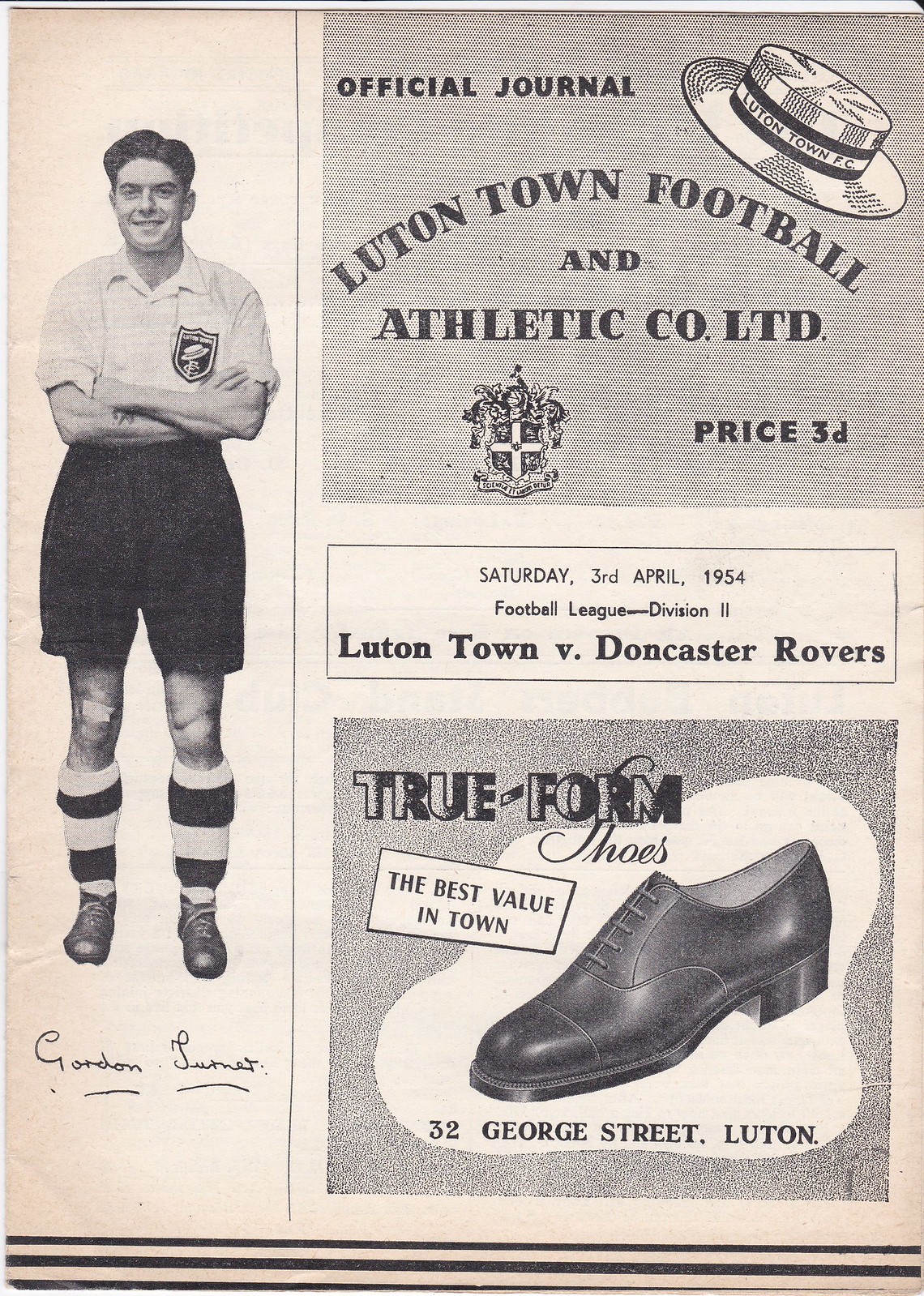The image is an old black-and-white photograph capturing a historic page from a sports magazine, specifically from the Lutontown Football and Athletic Company Limited. The left side features a detailed pane showing a male athlete in a rugby or soccer outfit, characterized by his big baggy black shorts, a white t-shirt with rolled-up sleeves, long socks, and cleats. His name, Gordon Lumet, is underlined below his figure. To the right, the image contains multiple sections: at the top, it reads "Official Journal, Lutontown Football and Athletic Company Limited" along with the price, marked as 3D. An emblem resembling a shield sits next to this text, accompanied by a picture of an old-fashioned straw hat labeled "Lutontown FC." Below that, another box indicates the match details: "Saturday 3rd, April 1954, Football League Division 2, Lutontown vs. Doncaster Rovers." At the bottom of the image, there is an advertisement for True Form Shoes, claiming to offer "the best value in town" and providing an address at "32 George Street, Luton." The overall aesthetic emphasizes a nostalgic, grayscale tone, characteristic of vintage posters or pamphlets.